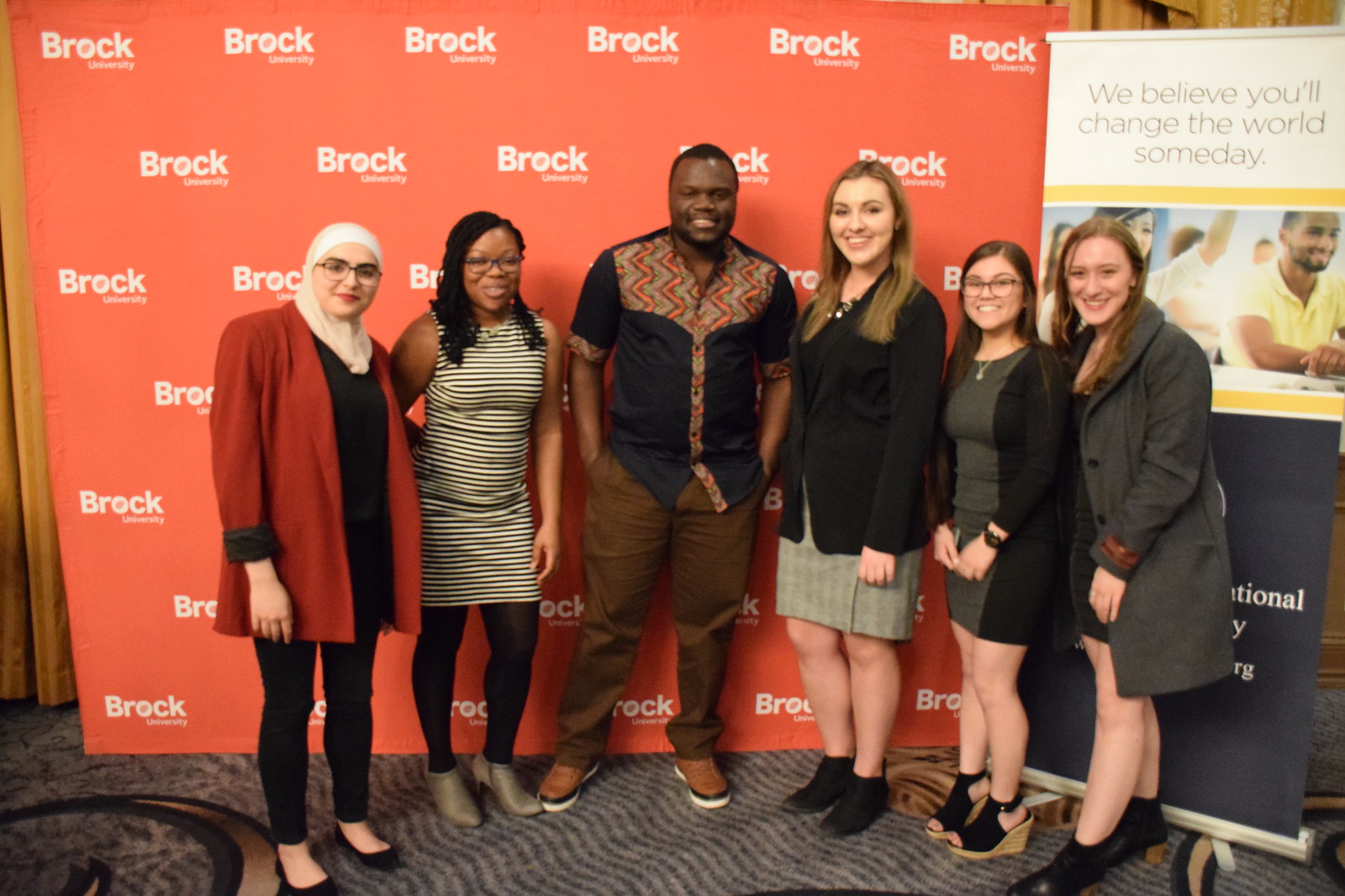This detailed photograph captures a diverse group of individuals posing together in front of a red background adorned with the words "Brock University" repeated in a grid-like pattern. From left to right, we see a Muslim woman wearing a white hijab, a red suit jacket, black pants, and black ballet flats. Beside her stands an African-American woman dressed in a white and black striped dress, paired with black stockings and silver shoes. An African-American man is also pictured, sporting a collared button-down short-sleeved shirt with an orange zigzag pattern, brown pants, and light brown shoes. There is a Caucasian woman in a black suit jacket, gray skirt, and black booties. Additionally, two other women can be seen in the background. On the right side, a white placard reads, "We believe you'll change the world someday," and features an image of people in a classroom. The carpet below them has alternating light and dark wavy lines, adding to the dynamic setting of the scene.